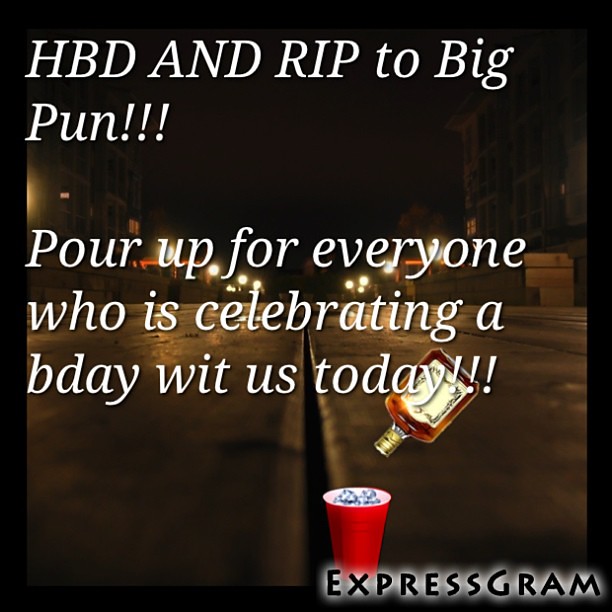The advertisement for Expressgram captures a vibrant nighttime city street scene, taken from a camera resting at street level, looking down the road. Illuminated by glowing street lights, the street features a rail line with buildings lit sparingly on either side. Atop this backdrop, bold text in black with a faint white drop shadow announces, "HBD and RIP to Big Pun!!! Pour up for everyone who is celebrating a B-Day with us today!!!" Accompanying this text is a hand-drawn graphic of a tilted brown liquor bottle, poised above a red Solo cup filled with ice, suggesting a celebratory toast. The Expressgram logo, also in black and capital letters with a subtle white shadow, is situated in the bottom right corner, completing the festive and commemorative scene.